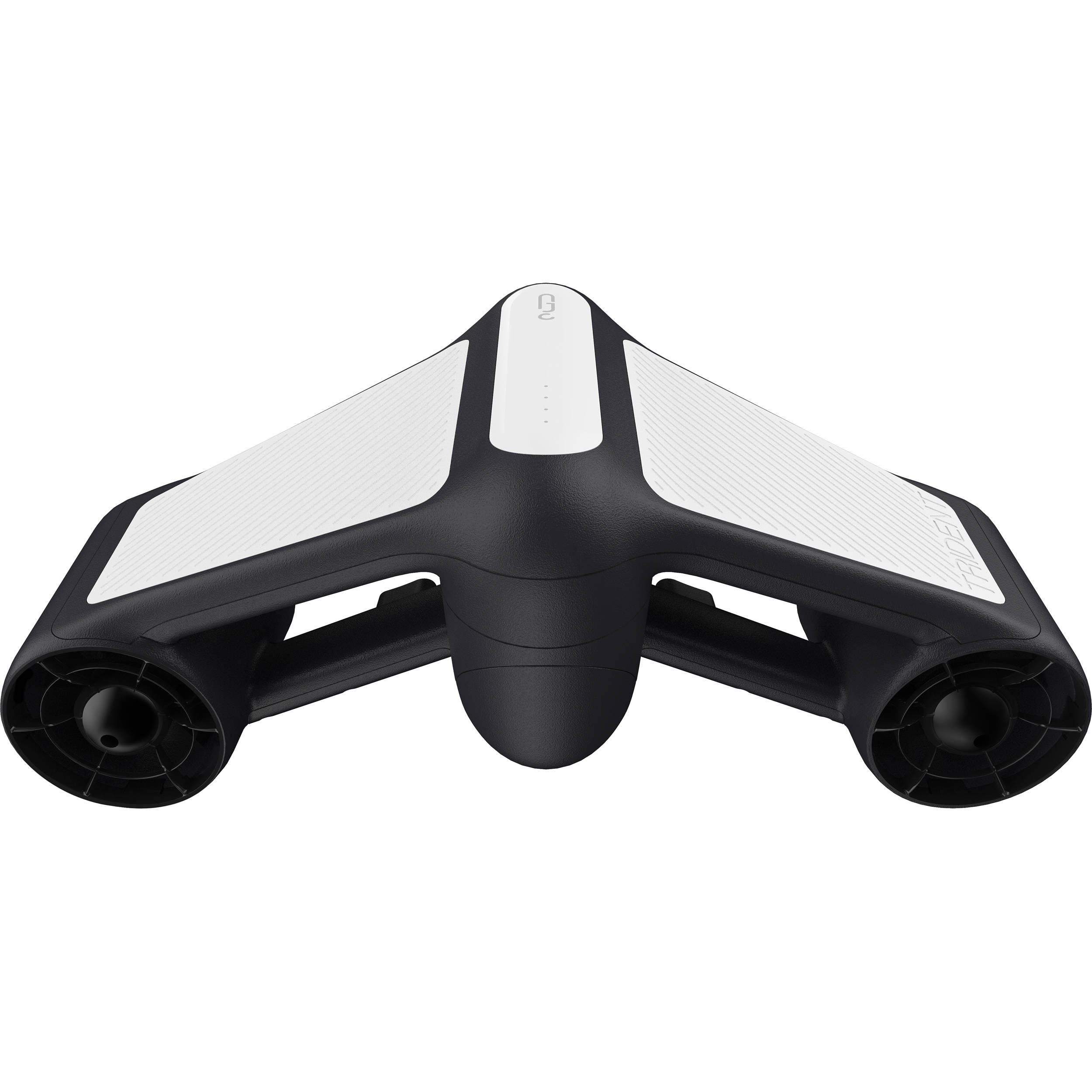The image shows a distinctive black and white drone, featuring a sleek and modern design. The drone's main body, crafted from dark black plastic, includes a sloped apparatus that resembles two ramps converging at a central piece, creating a seamless connection. This centerpiece is complemented by elongated trapezoidal triangles on both sides, which are white with black striping, adding a sophisticated contrast.

Underneath the main sloping sections, there are additional smaller ramps that contribute to the structural integrity of the drone. These black sections encompass cylindrical chambers housing fan-like apparatuses, each designed with a plastic sequenced structure comprising six interconnecting pieces. This intricate design mirrors itself on both sides of the drone, indicating a balanced mechanism for lift and stabilization.

The top of the drone features a small white panel, likely serving as the control console, situated atop the central black piece. This section, together with the elongated shapes on the drone, creates a compressed V-shape aesthetic that enhances the overall aerodynamic profile. Additionally, the left side of the drone bears a design element resembling a trident, while the center displays an elongated circular shape marked with a 'G' and an upside-down question mark in white. This area possibly indicates the branding or specific model information of the drone.